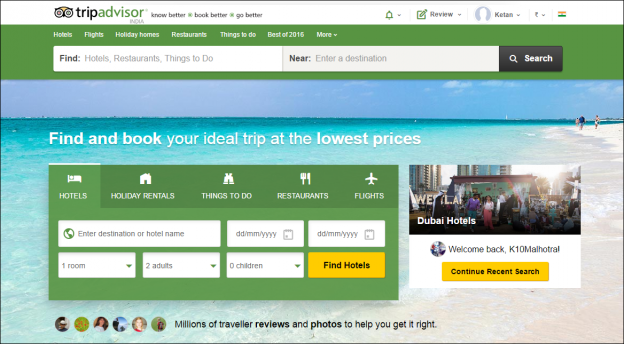This descriptive caption summarizes the image effectively and in detail:

---

The image is a horizontally oriented web screenshot of the TripAdvisor website. At the top, a white banner displays the TripAdvisor icon and name, accompanied by the slogan, "Know Better, Book Better, Go Better." To the right of this slogan reside a bell icon, a review notification, and the user profile name "Khitan," adjacent to which is an arrow and a small country flag icon.

Below this section, a green banner spans across the screen with two search boxes labeled "Find" and "Near," accompanied by a search icon. Directly beneath, a series of category headings include "Hotels," "Flights," "Holiday Homes," "Restaurants," "Things to Do," "Best of 2016," and more options.

The main content area of the screen features an eye-catching, light blue beach backdrop. A few figures are seen strolling along the shore, while gentle waves roll in on the right side. The sky is a light blue, complementing the scenic beach.

Overlaying this background are two text boxes. The first reads, "Find and Book Your Ideal Trip at the Lowest Prices." Below this is a green pop-up box containing selectable search categories: "Hotels," "Holiday Rentals," "Things to Do," "Restaurants," and "Flights."

To the right of the search box is an advertisement for Dubai Hotels, featuring an image of people in Dubai. Beneath the ad, the text warmly welcomes the user, "Welcome Back Khitan Malhotra," followed by a yellow button labeled "Continue Recent Search."

In the lower left quadrant of the image, six small profile pictures are displayed, accompanied by the caption in small black text: "Millions of Traveler Reviews and Photos to Help You Get It Right." The entire web page screenshot is outlined by a very thin black border.